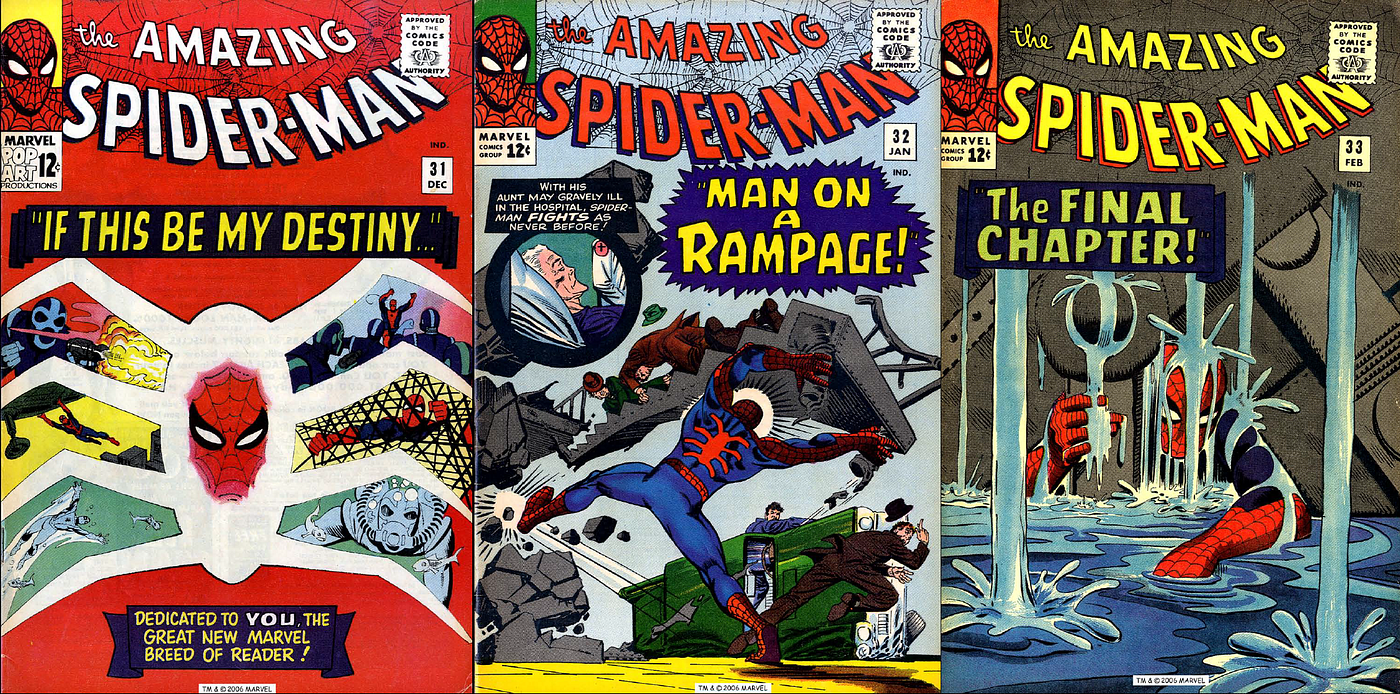Displayed in a rectangular poster, we see three side-by-side covers of "The Amazing Spider-Man" comics from issues 31 to 33. Each cover boasts distinct and vivid artwork:

The first cover, set against a red background, features a prominent white outline of a spider, with Spider-Man's red-masked head at its center. Inside the spider's body are scenes from the comic, hinting at the storyline within. At the top, bold white letters spell out "The Amazing Spider-Man," and a yellow box in the top left corner contains Spider-Man's head. A blue banner at the bottom, bearing yellow text, reads, "Dedicated to you, the great new Marvel breed of reader."

The second cover, action-packed with a blue backdrop, depicts Spider-Man in a dynamic pose, ripping a large piece of concrete with his back facing the viewer. There's a tipped-over green truck in the background, along with people reacting to the chaos. The title "The Amazing Spider-Man" appears at the top in red, against a webbed background. In the top left corner, a small green box showcases Spider-Man's head, and a blue banner below the title declares, "Man on a Rampage," in yellow.

The third cover has a gray-toned background, illustrating Spider-Man in a perilous situation, seemingly trapped in a flooding room with metallic walls. He clings to a metal pole with water splashing around him, possibly in a sewer setting. The comic's title shines in yellow at the top, with a nearby red box containing Spider-Man's head. Below the title, a blue banner with greenish text announces, "The Final Chapter."

Each cover vibrantly captures the essence of Spider-Man's adventures and the dramatic stakes of the narratives enclosed within these classic comic issues.